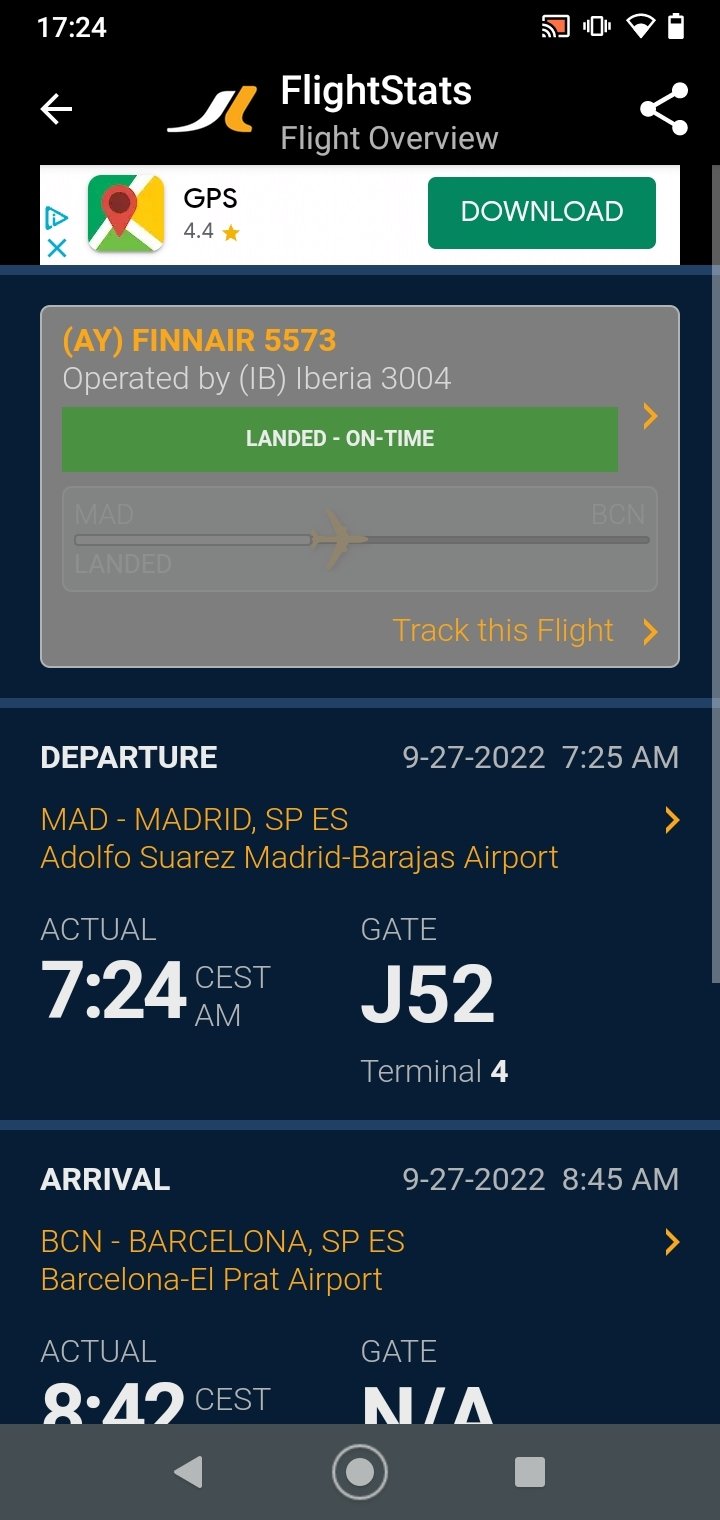Image Caption: Detailed Tracking Screen of AY Finnair Flight 5573

The image displays a vertically aligned smartphone screen featuring a flight tracking interface. The screen has a black background and contains various informational and interactive elements.

**Header:**
- **Time Display:** The top right corner shows "17:24," which appears to indicate the current time.
- **Icons:** Adjacent to the time are several symbols: a red Chromecast button, a phone icon flanked by two lines (probably indicating network strength or connection status), an internet connectivity symbol, and a battery symbol.

**Flight Information Section:**
- **Title and Logo:** Below the header, the text "Flight Stats" and "Flight Overview" is displayed alongside a logo resembling the letters "J" and "L."
- **Navigation Icons:** A left-facing arrow is situated on the left side of this section, and a triangle with dots is on the right side.

**Flight Details:**
- **GPS Data:** The text "GPS 4.4 download" appears, accompanied by a green button.
- **Flight Number and Status:** The flight information reads "AY Finnair 5573 operated by IB Iberia 3004," followed by the status "Landed and On Time." An orange arrow is positioned to the right of this text.

**Tracking Feature:**
- **Tracking Icon:** Below the flight status, there is a small airplane icon, typically used for flight tracking interfaces.
- **Tracking Link:** The text "Track this flight" is displayed in orange, with an arrow pointing left.

**Timings:**
- **Departure and Arrival Times:** The bottom section provides details on the flight's departure and arrival times, relevant to AY Finnair Flight 5573.

Overall, this screen offers a comprehensive overview of the aforementioned flight, including status updates, important symbols, and navigational features for further tracking, tailored for a mobile user.